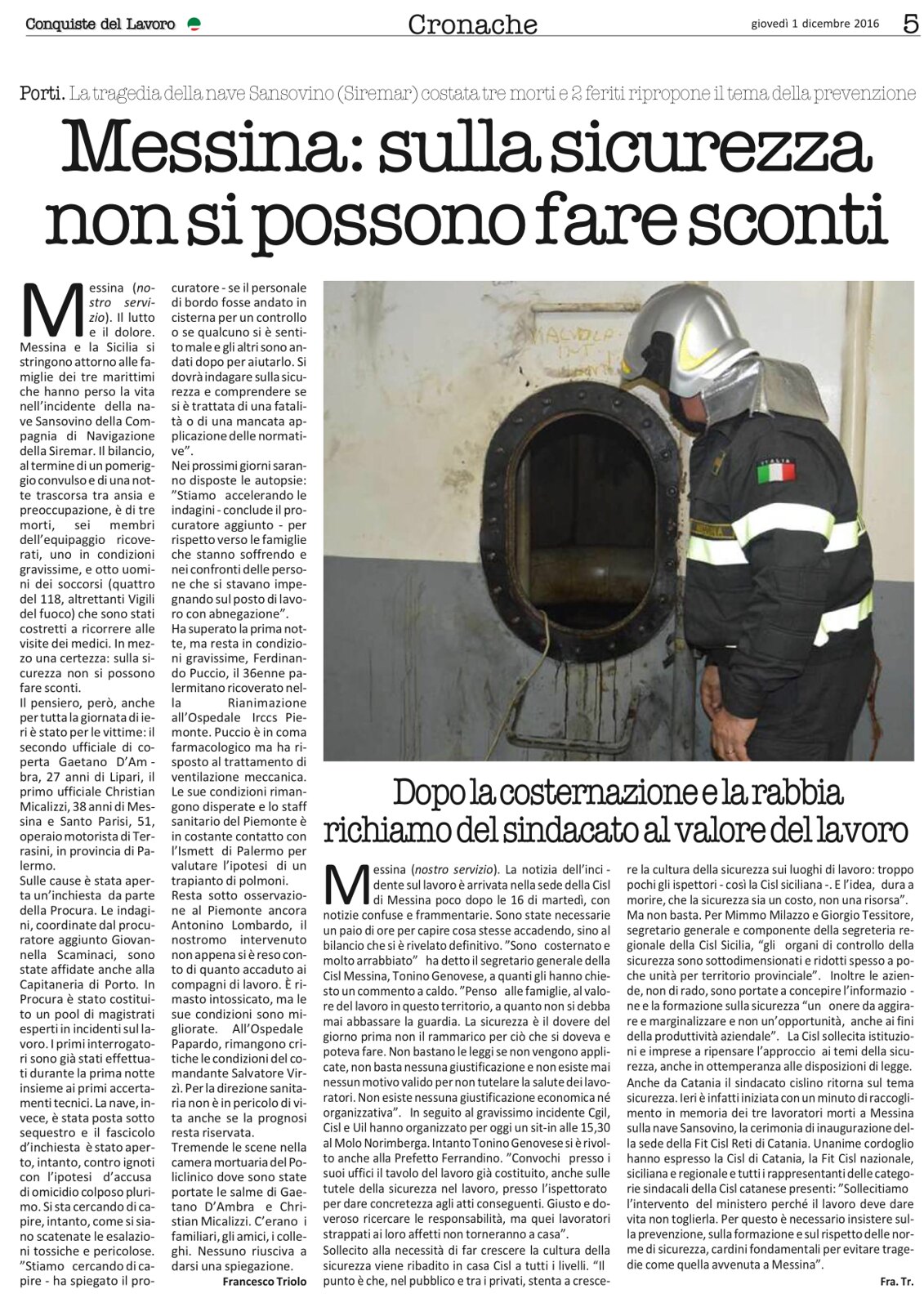The image depicts a page, possibly a clipping from an Italian newspaper or magazine, featuring a formal article against a white background. At the top left, the publication's title reads "Conquista del Lavoro," while the center headline states "Cronache." The top right displays the date "Giovedì, 1 December 2016" and the number "5," indicating it might be the fifth page of the publication. A prominent headline in bold reads "Messina: Sulla sicurezza non si possono fare sconti." The article is composed of dense, small print.

Towards the right half of the page is a photograph of a uniformed man, viewed from the left. He wears a black outfit with white reflective stripes on the arm and waist, an Italian flag patch on his shoulder, and a grey, silverish helmet. The man appears to be inspecting a small, oval window-like opening, possibly on a ship or within an industrial setting. The overall scene suggests a focus on safety inspections or regulations.